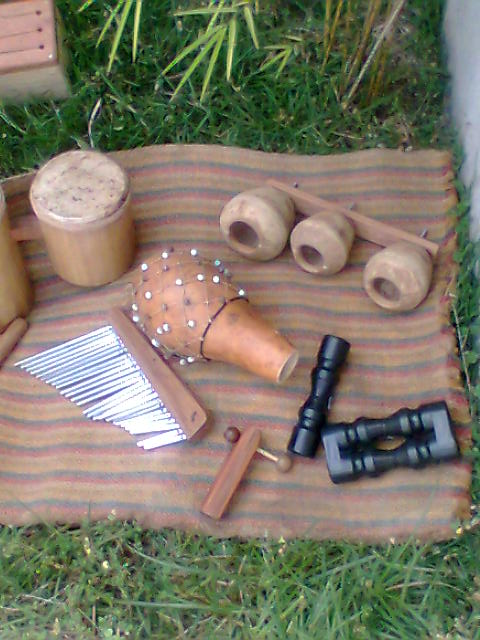The image depicts a woven fabric placemat with horizontal stripes of blue, red, beige, and brown, laid on short green grass. Arranged meticulously on the placemat are various earth-toned musical instruments from different cultures, suggesting a rustic and eclectic collection. In the center, there is a round drum with a brown barrel body, topped with stretched animal skin. Laying prominently on the drum is a gourd shaker adorned with netting and beads, likely from African or Latin American origins. To the lower right, a wooden stick with multiple hanging wind chime pipes is featured, likely creating a melodic sound when agitated. Additionally, there is a peculiar wooden piece with three attached pots, assumed to produce varying tones when struck. Lastly, a small circular container with an ivory and brown marble lid and a mysterious pipe-like tube with an unknown function are among the displayed items. Together, these objects present a harmonious blend of cultural artistry and musical diversity.